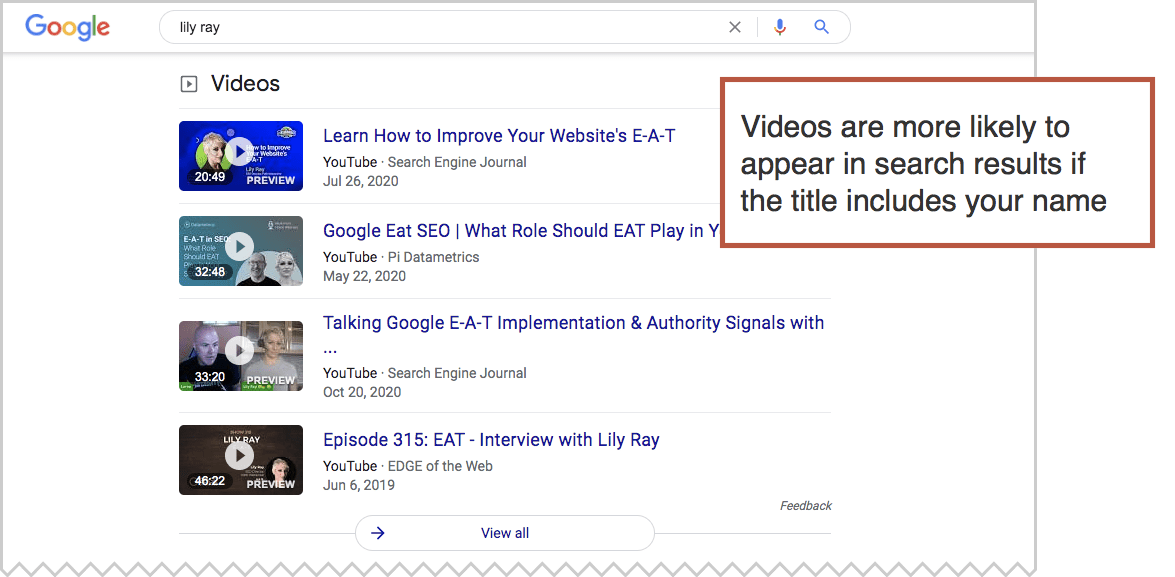An image under the category of websites captures a Google search interface. The prominent Google logo sits above a search bar containing the text "Lily Ray," accompanied by a microphone icon allowing for voice-to-text input and a magnifying glass icon to initiate the search. A red box highlights an informative statement in the upper right corner of the screen: “Videos are more likely to appear in search results if the title includes your name.” Below the search bar, a section labeled "Videos" displays various video results. The first video, titled "Learn How to Improve Your Website's EAT," features a thumbnail image of a woman. The following entry, "Google EAT SEO: What Role Should EAT Play?" showcases a thumbnail with two figures, one of which appears to be an artificial robot in the background with a man in the foreground. Additional listings include "Talking Google EAT Implementation and Authority Signals" and "Episode 315: EAT Interview with Lily Ray."